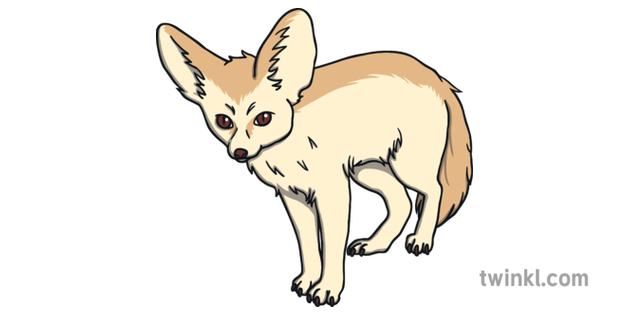This is an animated or computer-generated image of a small fox-like animal. The background is entirely white, and the focus is solely on the animal, which is standing and facing at a downward angle to the left. The creature has a light brown body with a slightly darker brown running from the top of its head, down its back, and covering its fluffy tail, which is lowered in the picture. Its head is small and dog-shaped with large, pointy ears that are light brown on the outside and cream-colored on the inside. The eyes and nose are dark brown, and the lower half of the body and face have a cream color. The animal's nails are a deep brown. The image is relatively simple and low detail, yet it effectively uses lines to suggest fluffiness and hair texture. The text "twinkl.com" is displayed horizontally in gray at the lower right-hand corner of the image.